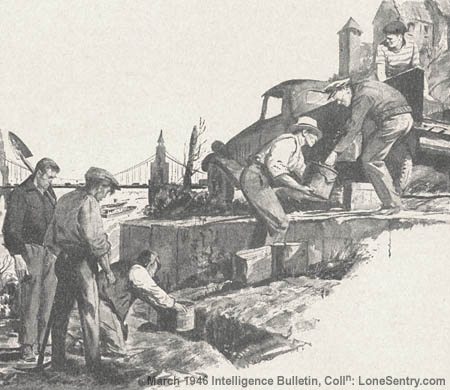This detailed black and white sketch, titled "March 1946, Intelligence Bulletin," and credited to LoneCentury.com, captures a vintage scene of six men engaged in what appears to be a construction or excavation task. The setting seems reminiscent of post-war Europe, possibly France, indicated by the architectural styles in the background, including a house and a distant bridge with a boat underneath.

The men are sprawled across three distinct levels of a small hill or trench area. At the base, three men are busy: one kneels to fill a medium-sized bucket, while the other two stand close by, one with a shovel over his shoulder, watching intently. Moving up a makeshift stair-step level, another man receives or passes a bucket. Further up, near the top level, stand two more men beside an old, period-appropriate pickup truck. One man is in the truck's bed, dressed in a white and black striped shirt and a derby hat, looking down at the workers. The other man, wearing white suspenders and a white hat, hands off a bucket.

In the background, beyond the busy scene, a house and a bridge over a river are clearly visible. The overall composition suggests a post-war effort, perhaps an engineering, construction, or repair project, with the men collaboratively passing buckets—possibly of soil or water—up the incline. The image exudes a vintage aura, emphasizing the collaborative human effort during the mid-20th century.